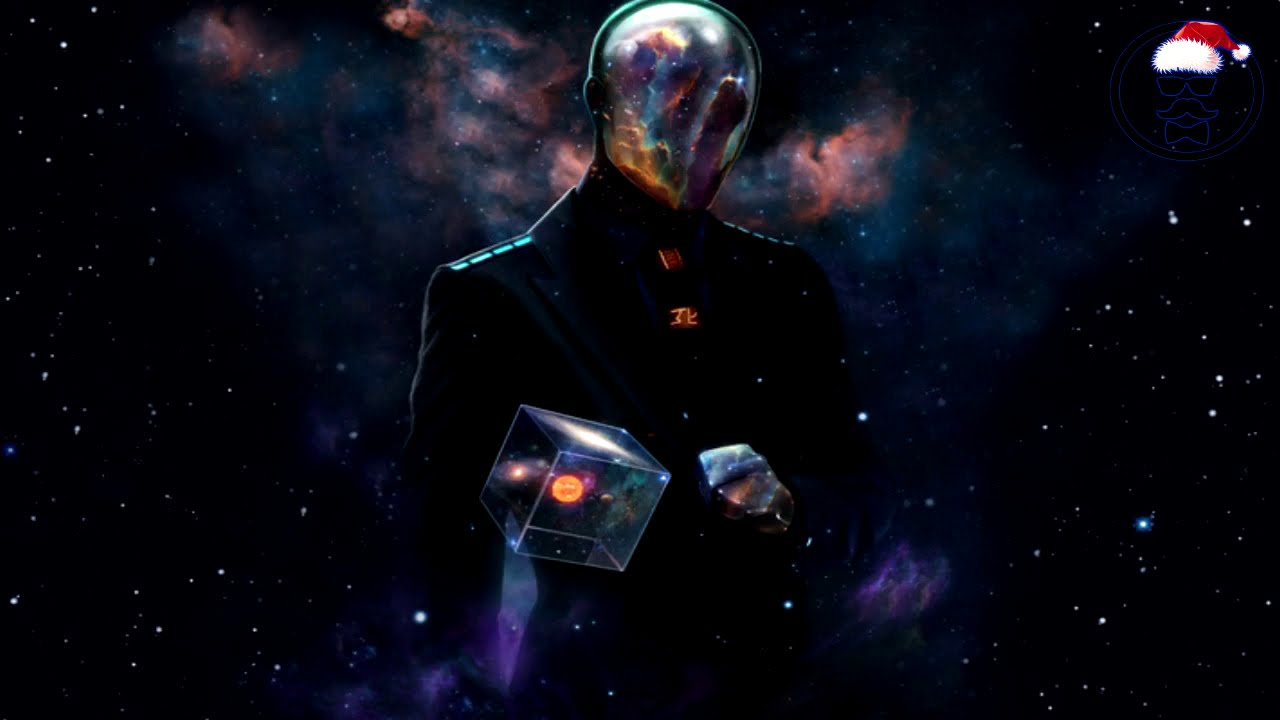The image depicts a surreal scene set against a dark, outer space backdrop filled with stars and vast nebulae, showcasing hues of black, blues, purples, and pinks. At the center stands a faceless man adorned in a black suit. Instead of a face, he has a mask that appears as a telescope lens reflecting the surrounding galaxies. His faceless head contrasts with his suit, blending seamlessly into the cosmic environment. Floating around his torso is a 3D cube exhibiting an array of galaxy colors—shades of orange, magenta, and dark blue—with an orange sphere or miniature sun inside it. The top right corner features a traditional red and white Santa hat, adding a whimsical touch to the space-themed composition. The overall atmosphere of the image exudes a cosmic, dreamlike quality, with no text to provide context or explanation.